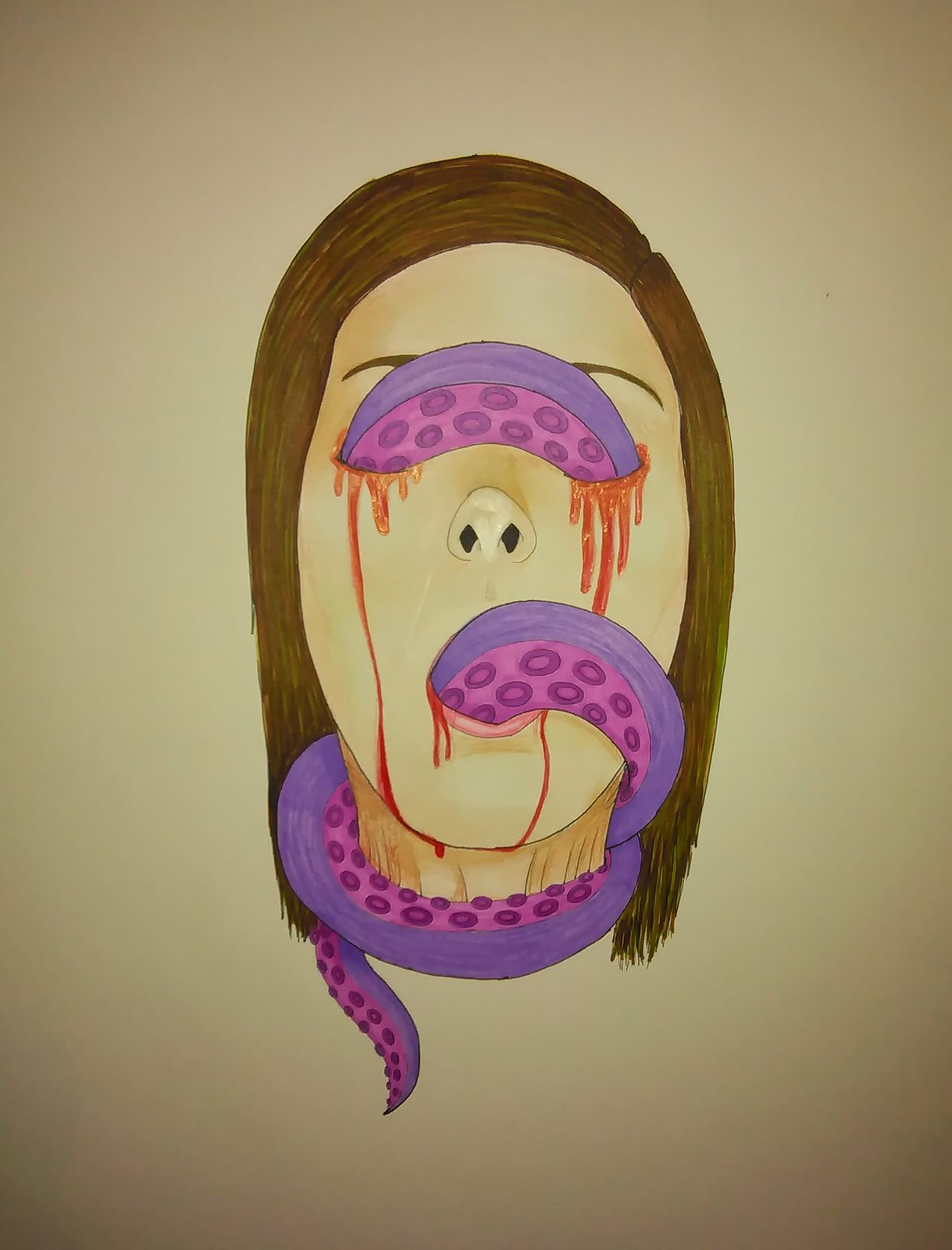This vividly colored drawing depicts a surreal, haunting image of a woman's face. Her long, dark hair cascades down to her shoulders, contrasting with her light skin. A striking feature of the artwork is a vibrant, purple snake that weaves through her eye sockets and mouth, wrapping itself around her neck. The snake's underbelly is a darker shade of purple adorned with what appear to be circular, suction cup-like patterns. The snake's tail extends past her neckline, tapering to a point.

Below her eyes, streams of red, yellow, and orange mimic the flow of blood, with similar hues trickling from the corner of her mouth, enhancing the eerie aesthetic. The drawing rests on a yellow or off-white sheet of paper, with dark gradients at all four corners that draw the eye towards the unsettling yet captivating central figure.